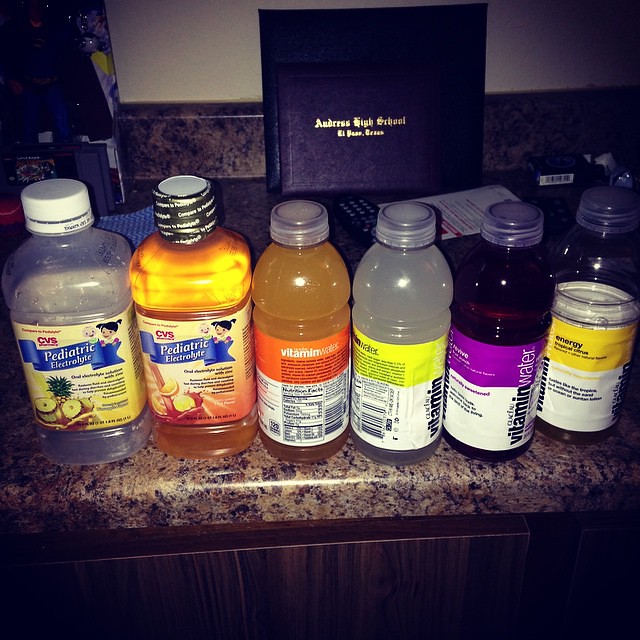The amateur close-up photo showcases a dark plastic laminate countertop, designed to mimic black and brown marble. Across the counter, there's a neatly arranged row of beverage bottles. Starting from the left, there are two CVS brand pediatric electrolyte drinks, one pineapple-flavored and the other of an unspecified flavor. Moving right, there are four vitamin waters: an orange-colored one, a yellow and white labeled one, a dark purple "Revive" flavor, and a tropical "Energy" variant. One of these vitamin waters appears half-drunk, possibly indicating regular consumption for nutritional reasons. The backdrop features a dark and slightly blurry area with a graduation-type booklet prominently displaying "Andrus High School." Other minor details include a TV remote, scattered papers, a box of cigarettes or gum, and a glimpse of a brown, fake wood grain cabinet door.